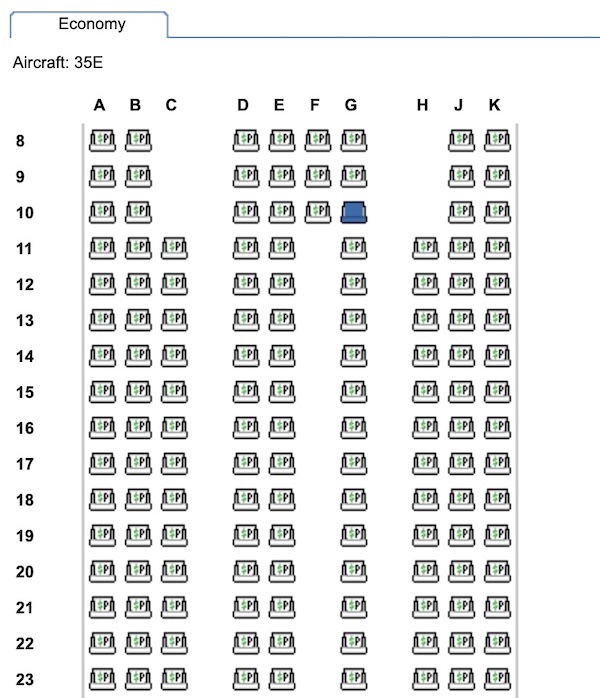The image illustrates the seating chart of an aircraft, specifically depicting the economy section. At the very top left, a tab labeled "Economy" is enclosed in a blue border that extends horizontally across the top of the page. Below this tab, the label "Aircraft 35E" is aligned to the left.

The top section of the chart displays column indicators for the aircraft seats, which are organized into three clusters marked ABC, DEFG, and HJK. These letters are presented in a black font. The left side of the chart lists the row numbers from 8 to 23.

Each row contains seat icons with letters and symbols, such as dollar signs and the letter "P." Notably, in rows 8, 9, and 10, seats are present only in columns A, B, J, and K. However, for the first three rows (8, 9, and 10), seats also fill columns DEF and G. From row 11 through to row 23, seating is available exclusively in columns D, E, and G.

A particular seat in row 10, column G is highlighted in navy blue, drawing attention amidst the other seating options. The detailed layout provides a clear and organized overview of the seat distribution within this section of the aircraft.